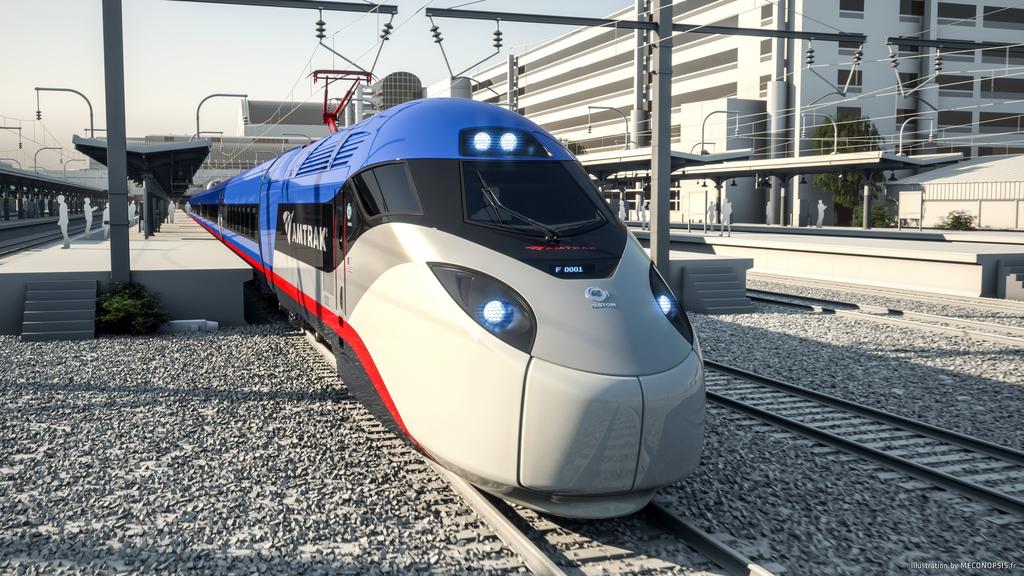This photograph features a sleek, high-speed Amtrak train captured from the front, prominently showcasing its modern design that resembles a snake with illuminated blue eyes. The front of the train is predominantly white, transitioning into a blue roof, followed by a sequence of color bands: a middle black section adorned with white "Amtrak" lettering, a wavy gray stripe, a straight red line, and another black stripe. The train possesses two headlights on its face and two additional ones on the top. The scene indicates a well-maintained station with new, clean gray platforms beside relatively new tracks, surrounded by gravel. The background reveals some gray figures on the platform, possibly embarking or disembarking. To the right, there is an empty lot and a substantial building, likely four or five stories high, that might be a parking garage or another structure. Electrical cables run overhead, hinting at the train's electrification. The overall atmosphere suggests that the train is preparing for departure, embodying both sophistication and speed.